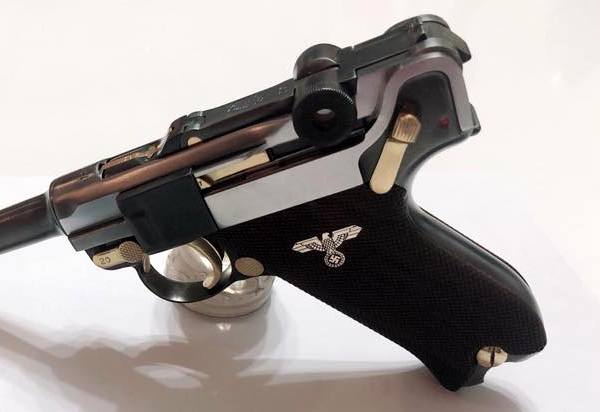This photograph features a vintage German handgun of unknown make, prominently displaying an eagle holding a swastika on its black grip, indicative of its Nazi association. Positioned at an angle, the gun is supported by a small silver metal stand, casting a shadow beneath it on a glossy white background. The gun is oriented with the barrel pointing down to the bottom left, partially out of frame. The firearm's top is constructed from polished steel with a visible copper stripe running across it. Several parts of the gun, including the trigger and safety, are crafted from gold, while other components such as fasteners are made from brass or bronze. Additionally, there is a distinctive "20" marking in gold on the gun, and a screw is noticeable at the base of the handle.